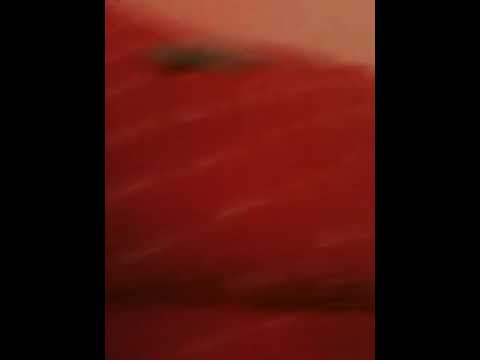The image features a blurry, vertically framed design that is difficult to discern. On either side, there are thick black borders occupying about a quarter of the image's width. The central portion displays a red to maroon background with various shades and textures, including lighter diagonal streaks. The top section of the image shows a pale beige or peach color, transitioning into the red area where a dark, indistinct streak crosses the bottom. Overall, the image evokes an abstract or artistic style, making it challenging to identify any specific objects or details due to the poor resolution and motion blur.